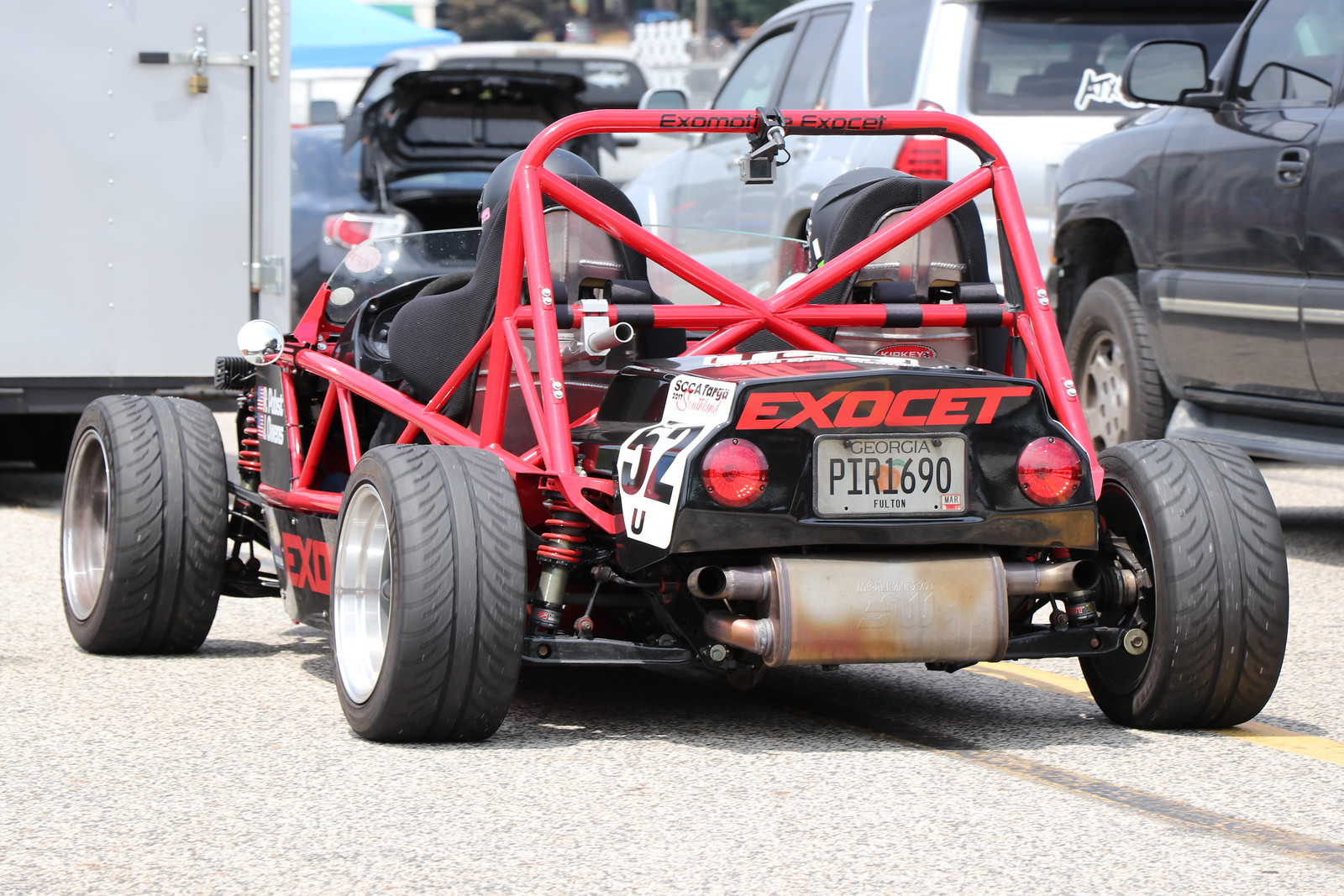The photograph captures an asphalt road, possibly a highway or an in-town road, marked by a yellow line running from the bottom right-hand corner diagonally to the left. Dominating the center of the image is a distinctive, street-legal race car resembling a dune buggy, characterized by its striking fire engine red frame and roll bars. This vehicle, lacking fenders, prominently displays a small black area above the engine, emblazoned with "EXOCET" in red. Above the Georgia license plate “PIR-1690,” a card with the number 52 hangs from the back left side.

The race car is positioned facing slightly to the left, allowing a partial view of its left side, where two horizontal red bars and additional vertical bars are visible. It features a small windshield, wide new tires with deep treads, and red shocks with matching red coils. Behind the race car, a white truck is visible towards the top left of the photograph. Additionally, a line of cars occupies the next lane on the right side of the image, contributing to the sense of traffic and movement.